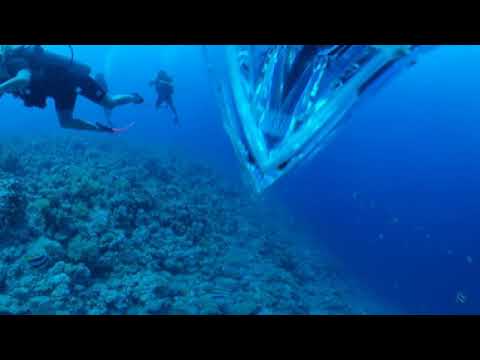This underwater scene features two scuba divers in the top left quadrant. The foremost diver, positioned horizontally, wears a black scuba outfit, with their legs pointed out and arms slightly bent forward. Behind this diver is a second one, more vertically inclined with arms extended in front. Beneath them stretches a seascape of coral and rock formations, swathed in hues of bluish-green, gray, and dark blues. Toward the upper right, an enigmatic object with a triangular-tipped, truncated form, almost diamond-like in shape, juts sharply downward. It appears transparent in parts, with dark and light blue tones accentuating its edges, giving it an almost crystalline, non-organic appearance. The background water transitions from dark blue in the depths to lighter shades near the surface, creating a vivid underwater tableau framed by subtle black borders at the top and bottom.